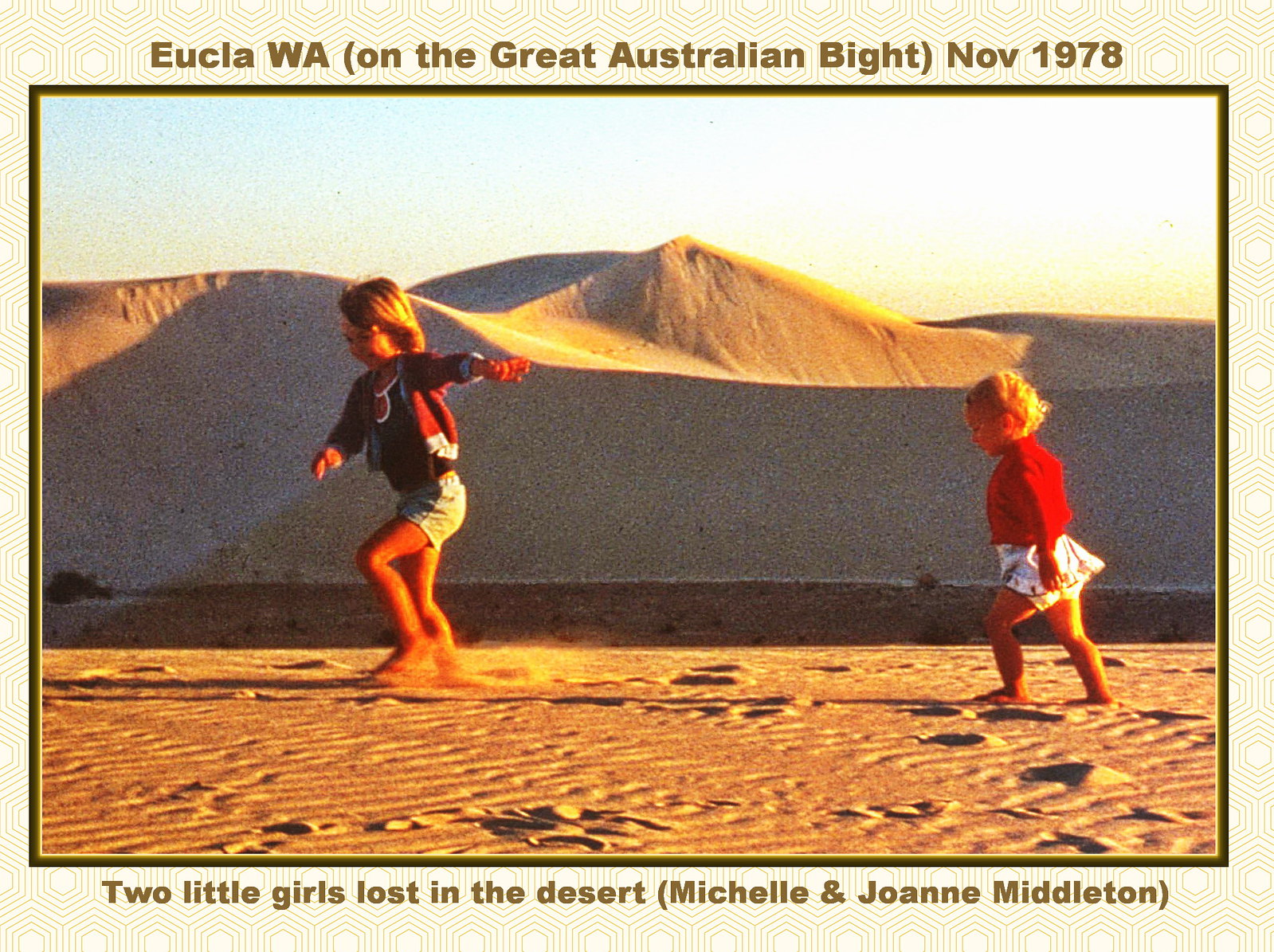The image depicts two young girls playing in a vast, tan sandy environment marked by large sand dunes that resemble mountaintops extending into the background. In the foreground, on the left, the older girl with blonde hair wears a red and white hoodie or sweatshirt over a black shirt with red accents and white or gray shorts. The younger girl beside her, also with blonde hair, is dressed in a red long-sleeve shirt and a white and black skirt. Both girls are barefoot, energetically kicking up the sand as they play. Above them, black text on a brown background frames the image, reading "Eucla, WA (On the Great Australian Bight), November 1978." At the bottom, brown letters on a white background state "Two little girls lost in the desert," with "Michelle and Joanne Middleton" noted in parentheses.